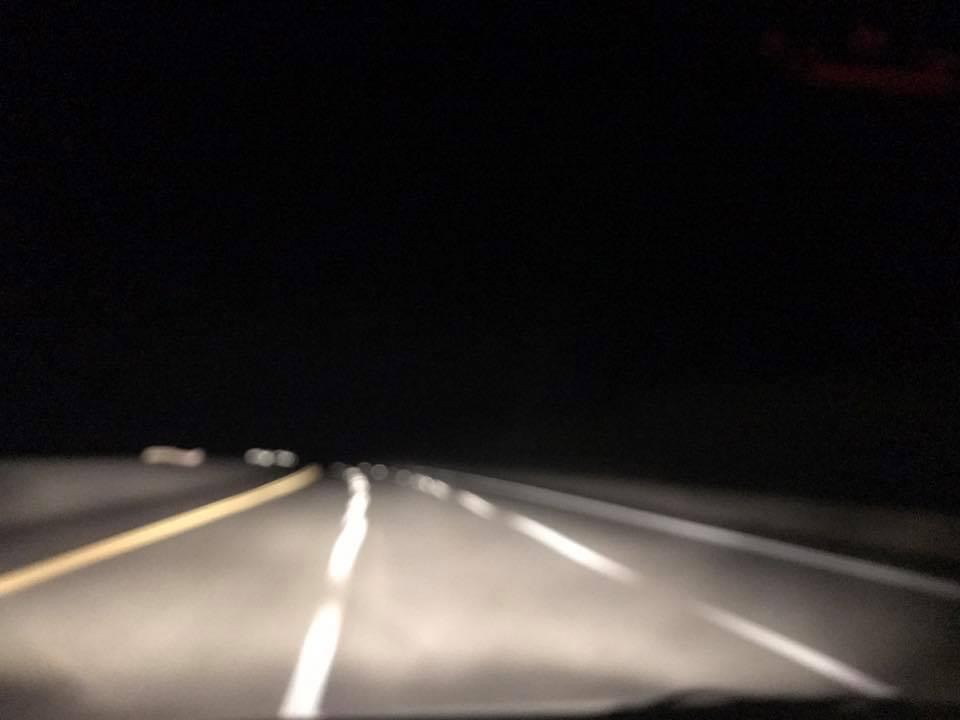A photograph captures the scene of a pitch-black night as viewed from inside a car, through the windshield. The image reveals a four-lane highway bathed in darkness, with only a faint strip of land visible on either side. In the far distance, the headlights of three or four vehicles approach, cutting through the enveloping shadows. The immediate foreground is heavily shrouded in darkness, with visibility extending only as far as the car’s own headlights, which cast a limited and dim glow on the road ahead. The overall atmosphere of the scene is one of isolation and mystery, defined by the inky blackness that dominates the surroundings.